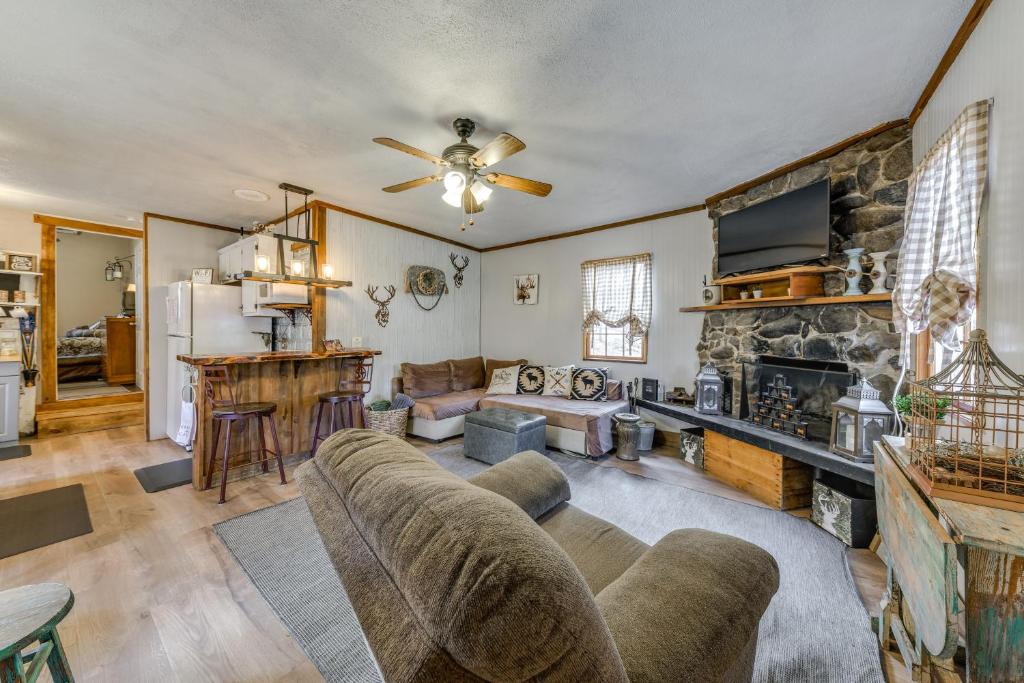The image captures an indoor photograph of a living room with a cozy, rustic design. The living room features white walls and ceilings, accented with exposed wooden edges that add warmth and character to the space. Dominating the right side of the room is a striking rock fireplace wall, topped with a wooden shelf that holds a flat-screen TV and some white vases. In front of the fireplace, a gray hearth is flanked by two lanterns, and a wooden storage chest sits at its base. 

A plush, brown recliner is situated closest to the viewer at an angle, providing a clear view of the TV. The floor is adorned with a light gray rug that complements the room's predominantly brown and earthy tones. To the left, an open kitchen area with a bar-style wooden countertop and a white fridge is visible, separated slightly from the living room. 

Central to the room, an L-shaped sofa with multiple throw pillows faces the fireplace, enhancing the living area's inviting atmosphere. A wicker birdcage is perched on a shelf table to the right of the fireplace. Above, a brown ceiling fan hangs in the center of the room, providing functionality and aesthetic appeal. The room is well-lit with multiple lights, making it feel bright and welcoming despite the abundance of wooden elements. 

Overall, the photograph captures a spacious and busy living area that seamlessly blends functionality with a cozy, rustic charm.